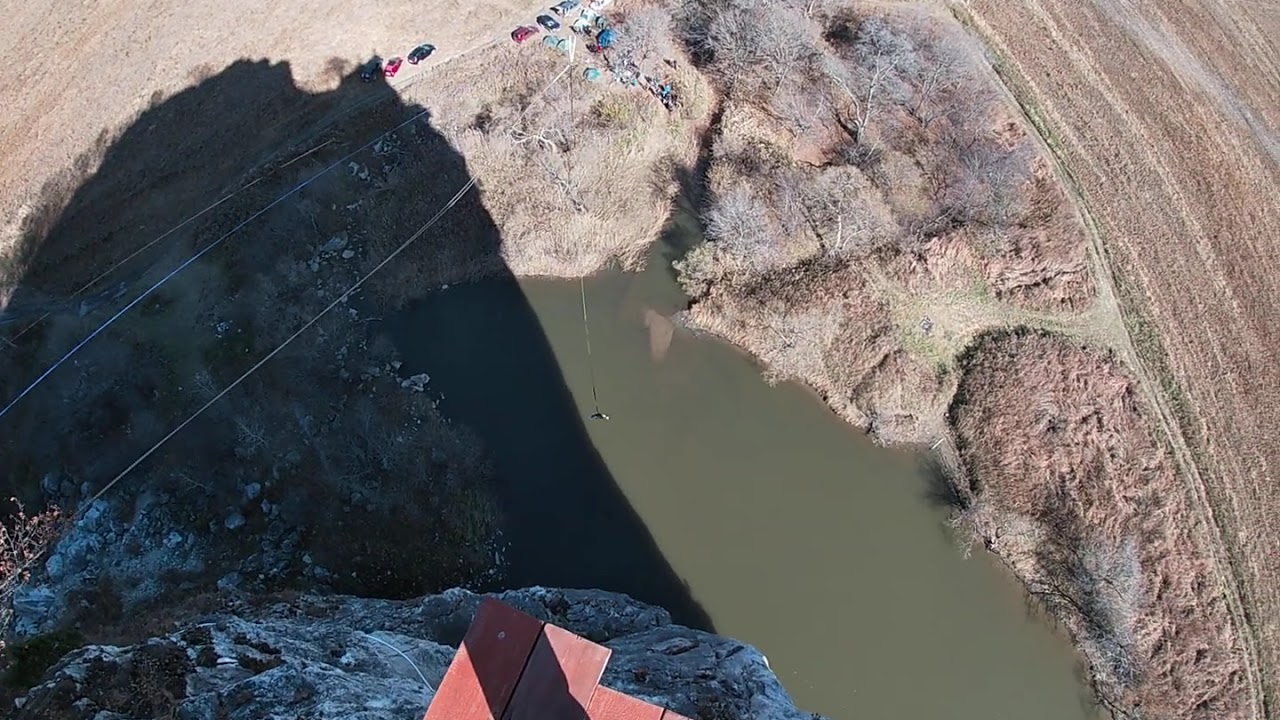The photograph captures a breathtaking aerial perspective from a high rocky cliff. The view looks down upon a landscape that includes a large, murky lake enveloped by faded grassy fields and scattered trees. The image also captures a sense of human presence with a small parking area featuring several cars—a blue car, two red cars, a white car—and a few people. Electrical wires or possibly zip line cables stretch from the top of the cliff towards the center of the frame. The scene is bright with ample sunlight, which casts a pronounced shadow of the vantage point—a prominent, stone-based structure or hill visible on the left side of the picture. In the mid-left, rocks and bushes can be seen, with the perspective showing off the rugged terrain. The lake’s water appears brownish-green, indicating a murky quality. A striking red platform is subtly visible near the bottom-center of the image, suggesting the viewpoint of the photograph. The overall environment looks dry and faded, with more brown hues dominating the scene, adding to the aged and weathered appearance of the landscape.